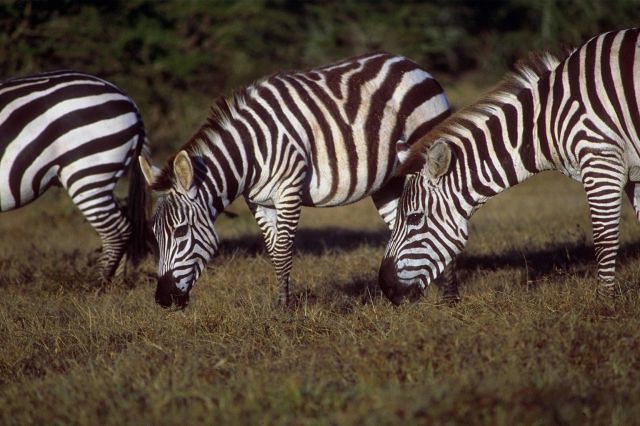In this exterior photograph taken in natural lighting, three zebras are the main subjects, standing in an open grassy area. All three zebras face towards the left side of the frame, creating a sense of alignment and continuity. The zebra on the left is only partially visible, showing its striped hindquarters and a long dark tassel on its tail. The middle zebra, partially obstructed, displays a prominent dark muzzle and eyes, with its head down, seemingly grazing. Its striking black-and-white striped mane stands short and upright. The zebra on the right, also grazing, has a thicker head and is visible only from the front half, which overlaps with the middle zebra. The entire scene is set against a backdrop of deciduous green vegetation, casting various shadows that add depth to the image. Despite their position, all zebras exhibit similar black-and-white stripes that extend down their bodies, contrasting against the lush grass and dense foliage behind them.